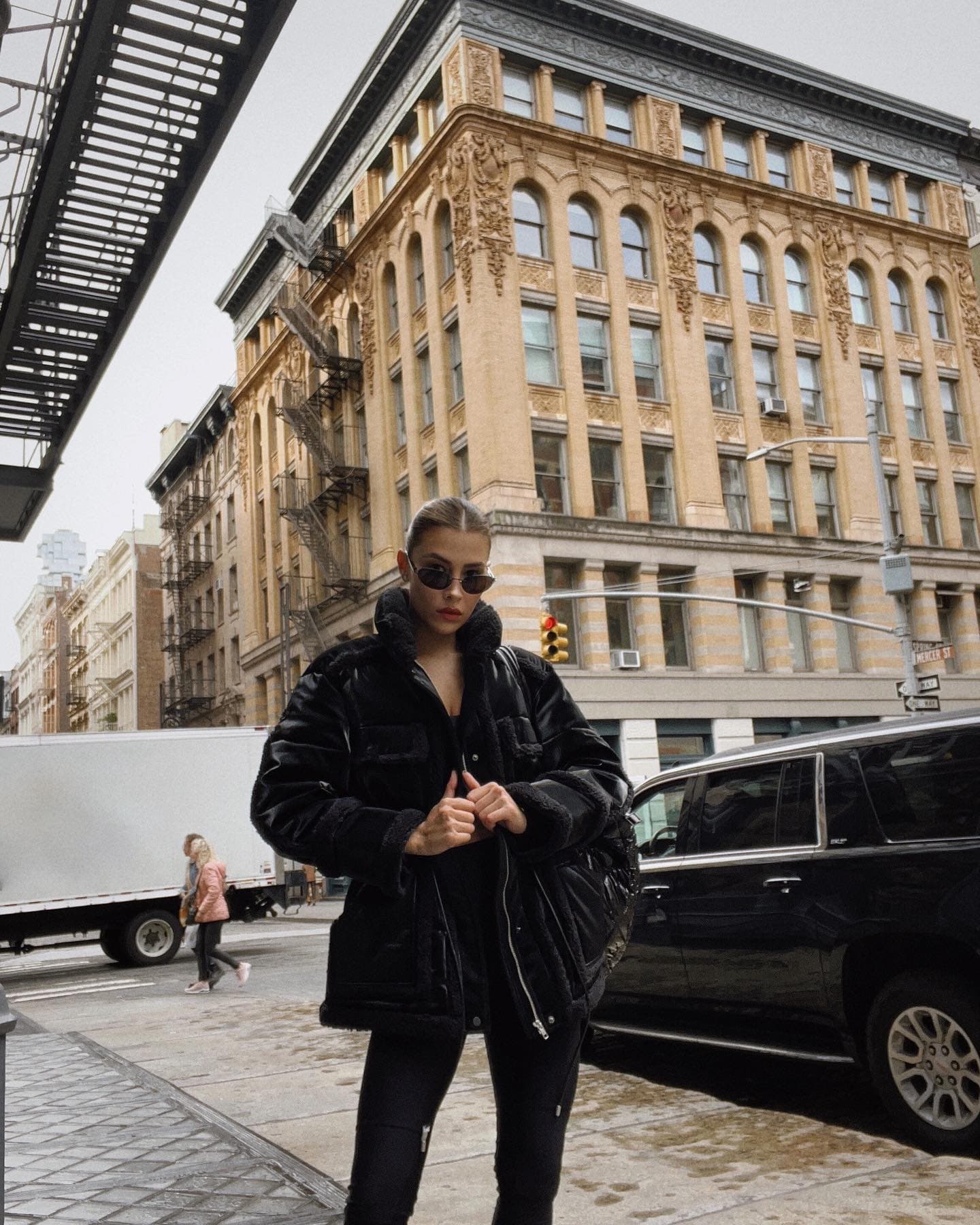In this striking fashion photograph, vertically oriented and set in a bustling downtown urban environment, a young Caucasian female model stands confidently at the lower center of the image. She exudes an effortless cool, wearing a distinctive fur-necked jacket zipped up to her bust line, her hands holding it closed just below. Beneath the jacket, she sports a low V-neck blouse, paired with sleek long black pants that add to her sophisticated ensemble. Her head is tilted downward, and she gazes over the top of her stylish sunglasses directly at the photographer, creating a captivating and slightly mysterious aura.

The urban backdrop adds depth and context to the scene. To the right of the model, a traffic light on a long metal support projects outwards, indicating the familiarity of city life. On the left side of the image, a small delivery truck can be seen moving through the intersection, accompanied by pedestrians crossing the street, bringing a sense of the ongoing daily bustle. Just behind the model to her left, a long black limousine is parked at the curb, subtly contributing to the urban elegance of the scene.

Dominating the background is an impressive six-story brownstone building with a flat roof and numerous vertical rectangular windows. The top floor features rounded arch windows, and a penthouse with a nearly square window tops off the structure. Fire escapes are visible on the building's left side, hinting at its age and character. This brownstone stands at the corner of the street, anchoring the photo in a quintessential city landscape.